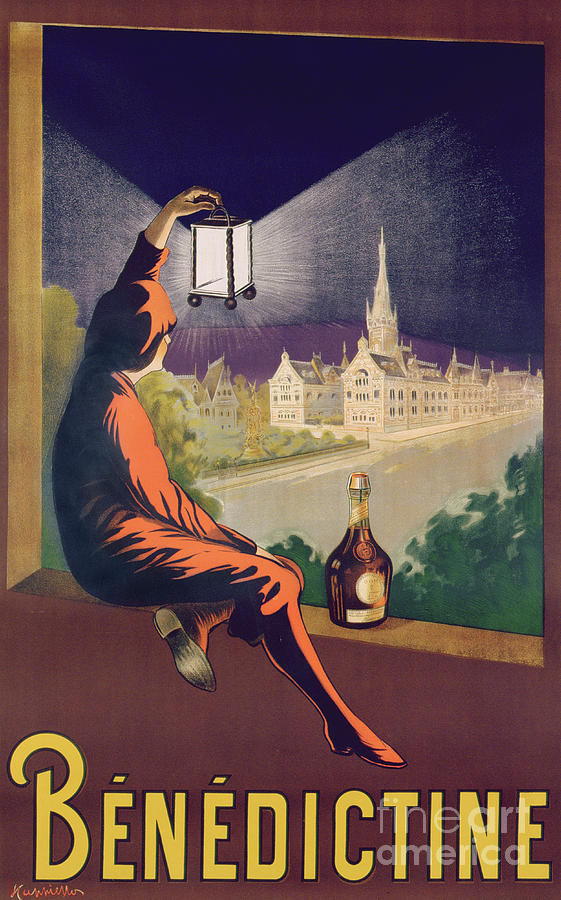This detailed hand-drawn artwork depicts a man sitting on a brown window sill, prominently wearing full-body red pajamas, complete with matching red shoes and a red cap. The man, positioned slightly to the left of center, is extending his left arm upward to hold a square lantern emitting bright white light in all directions except straight up. His right leg is extended forward, while his left leg tucks beneath his right. Beside him, on the window sill, rests an unopened wine bottle with a brown hue.

The scene outside the window reveals a nocturnal cityscape featuring a river that flows through the town. To the right of the river, we see a series of trees, while the left side showcases multiple buildings, including a notable church or cathedral with white and gold exterior details. The church features a prominent gold-and-black steeple topped with a cross. Nearby, additional structures, including what appears to be a statue in a courtyard and a blue skyscraper, complete the urban panorama.

At the bottom of the image, the word “Benedictine” is boldly inscribed in yellow with a black outline. In the bottom right corner, the watermark "Fine Art America" is displayed in small, semi-transparent white text.